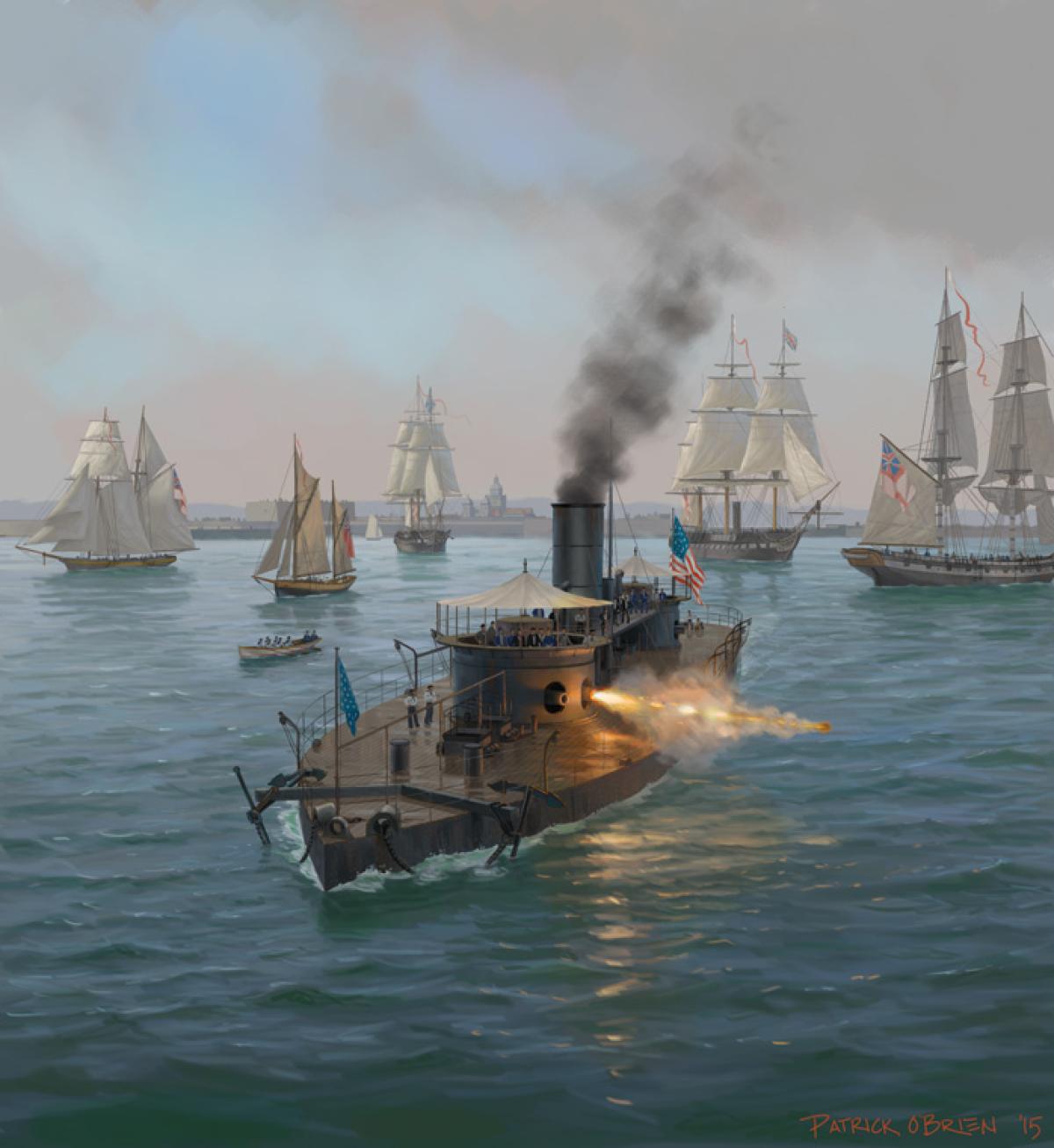This image appears to be a detailed painting, potentially by Patrick O'Brien, depicting a dramatic maritime scene. The central focus is a large, steam or coal-powered warship, which looks reminiscent of a Confederate type vessel from the 16th or 17th century, prominently featuring an American flag in red, white, and blue. The warship, gray in color, has a visible cannon actively firing a shot. Surrounding it, a serene yet somewhat turbulent body of blue water with gentle ripples hosts several other vessels, including traditional brown ships with white sails and a small canoe-like boat. The background fades into a distant cityscape, partially obscured by gray clouds interspersed with patches of blue sky. Notably, one of the background ships seems to bear a British flag, adding a historical international element to the scene. Overall, the painting captures a moment of historical naval activity with meticulous attention to color and detail.